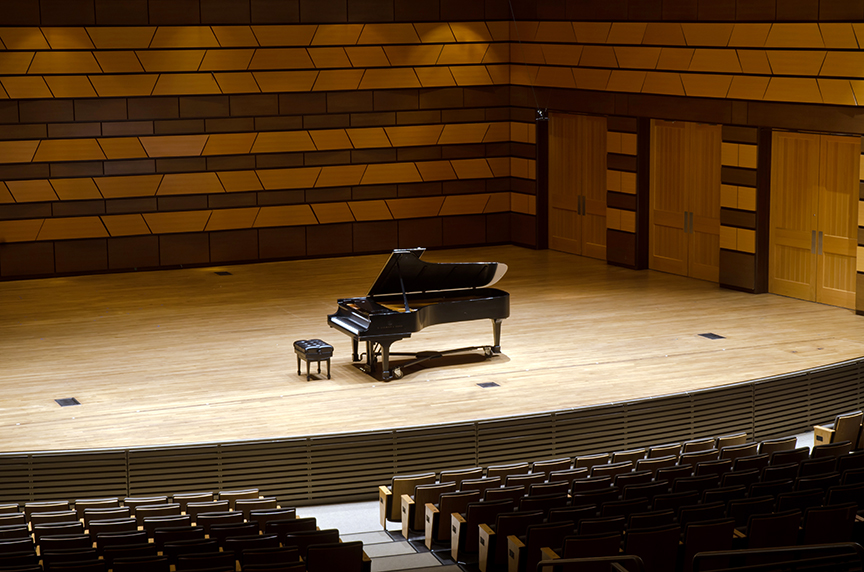The image depicts a large, empty music hall centered around a grand, predominantly light brown wooden performance stage. Positioned in the middle of the stage is an open black grand piano accompanied by a black leather stool set to the left. The stage is spacious and illuminated with focused lighting on the piano, casting it into brighter emphasis compared to the darker ambiance of the backdrop.

The backdrop features an intricate wood pattern, alternating between dark and light brown, with horizontal line segments interlaced with slanted lines, a design likely intended to enhance acoustical reflection. On the right side of the stage, three closed wooden double doors are visible. The hall is equipped with inclined seating, showcasing rows of chairs with wooden armrests and black leather seats, distinctly divided by a central aisle. Overall, the scene captures a purposeful mix of functionality and aesthetic in its design, ready to host a performance.